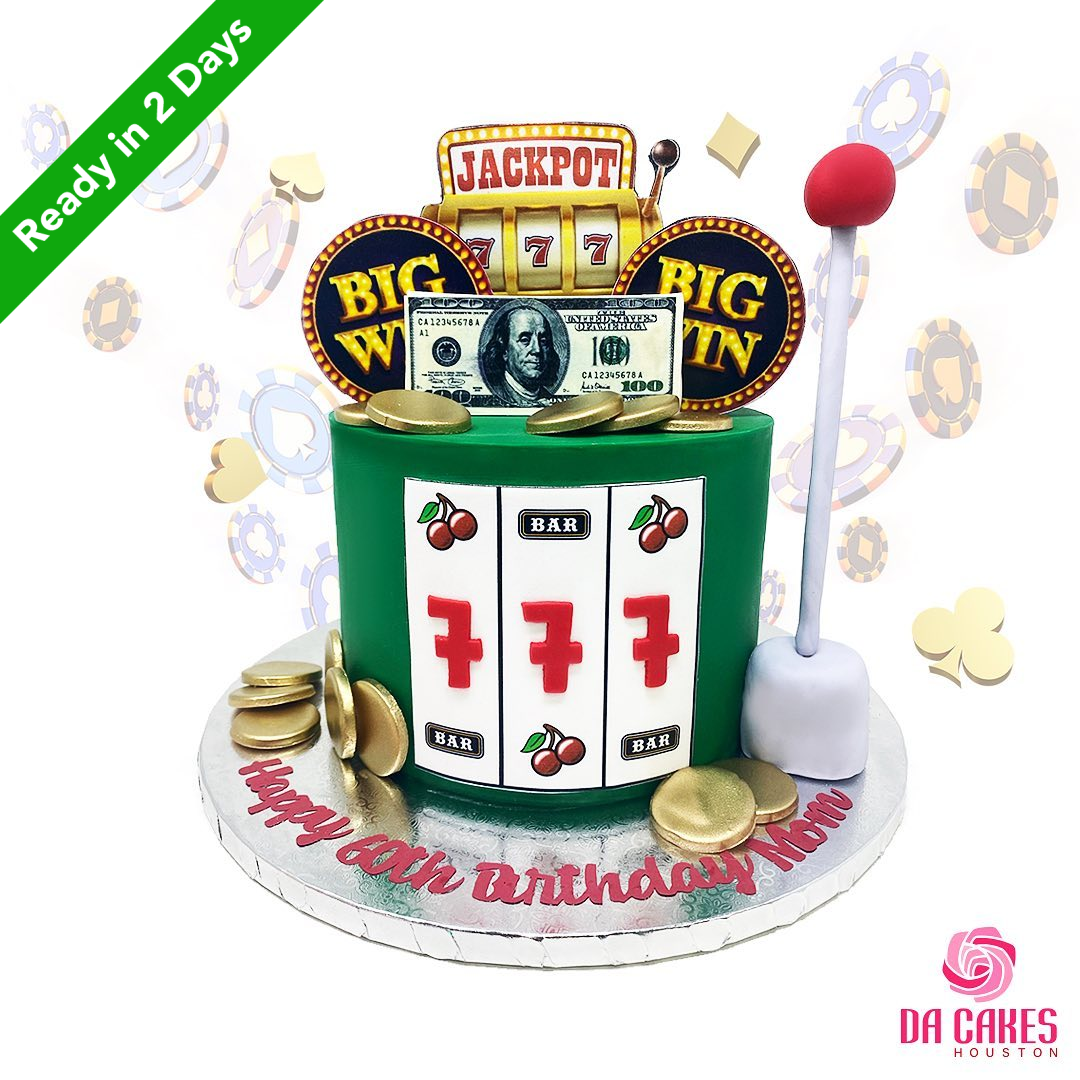This is an elaborate color advertisement for Duck Cakes of Houston, featuring a highly detailed, slot machine-themed cake. The background is filled with casino-themed decorations, including poker chips and three-dimensional icons for the four suits of a card deck. In the center of the image is a tall, round cake designed to resemble a slot machine, primarily colored green with silver foil accents. 

Atop the cake is a graphic party hat with a silver brim and a green top, adorned with an icon showing a jackpot of three red sevens. Below this, two large discs reading "Big Win" in gold letters on a black background are prominently displayed. In front of the cake are several representations of hundred dollar bills and gold coins, adding to the casino aesthetic.

The cake features intricate details such as a front panel designed like a slot machine with another set of triple red sevens on its reels, cherry icons, and bar symbols. Scattered around the hat's brim are additional gold coins, further enhancing the motif. On the right side of the cake, a lever modeled after a slot machine's handle features a red knob.

Celebratory text on the silver platter base reads "Happy 60th Birthday, Mom" in red cursive. In the top left corner of the image, a green banner with white text announces "Ready in 2 Days." The bottom right corner showcases the cake's creator with a pink rose icon and reads "Duck Cakes of Houston" (spelled D.A. Cakes).